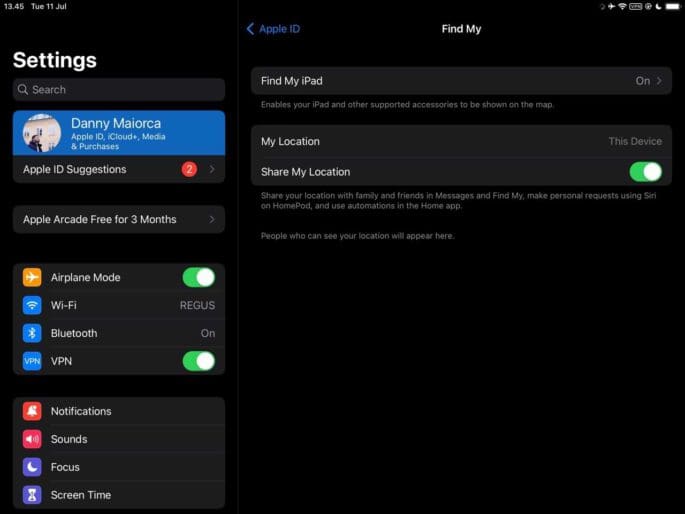The image depicts a smartphone screen with a black background. In the top left corner, the date and time are displayed as "Tuesday, 11 July, 13:45." The top right corner shows a full battery icon. Below this, on the left side, there is a section titled "Satin" in large white letters. Directly beneath this, a dark grey search bar with a magnifying glass icon is visible.

Further down, a blue rectangular section features a round profile picture on the left, and beside it in white text, it reads, "Danny Majorca, Apple ID, iCloud Plus, Media and Purchases." Below this section, there is a notification labeled "Apple ID Suggestions," marked with a red circle containing the number 2.

Moving further down, there's a dark grey box with a drop-down menu option, labeled "Apple Arcade, free for 3 months." Following this, a grey box displays an orange square with an airplane icon, indicating "Airplane Mode." This mode is turned on, as shown by a green-lit toggle bar shifted to the right.

Below the Airplane Mode setting, the screen lists "Wi-Fi" with a blue square next to it labeled "REGUS." Finally, at the bottom of this section, "Bluetooth" is indicated along with its standard icon.